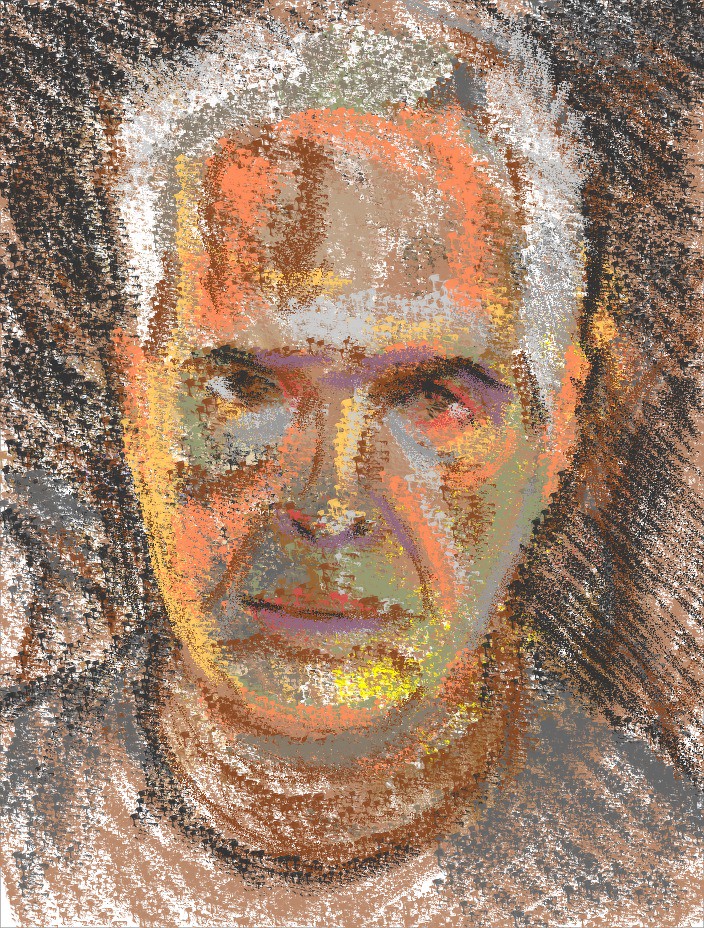The image portrays a close-up, chalk-style self-portrait of an older Caucasian man with short white hair, rendered with a splotchy and smudged technique. Despite the stylized approach and low detail, we can discern key features: the man has brown eyes, lines around his mouth indicating age, and is wearing a gray shirt with an orange turtleneck or scarf around his neck. The backdrop is a sketchy mix of dark brown, gray, and black, complementing the muted, primarily orange, yellow, and purple tones used in the portrait. The man's expression is neutral, with his mouth closed and his face slightly angled. Notably, there are no additional subjects or artist's signature in the image.